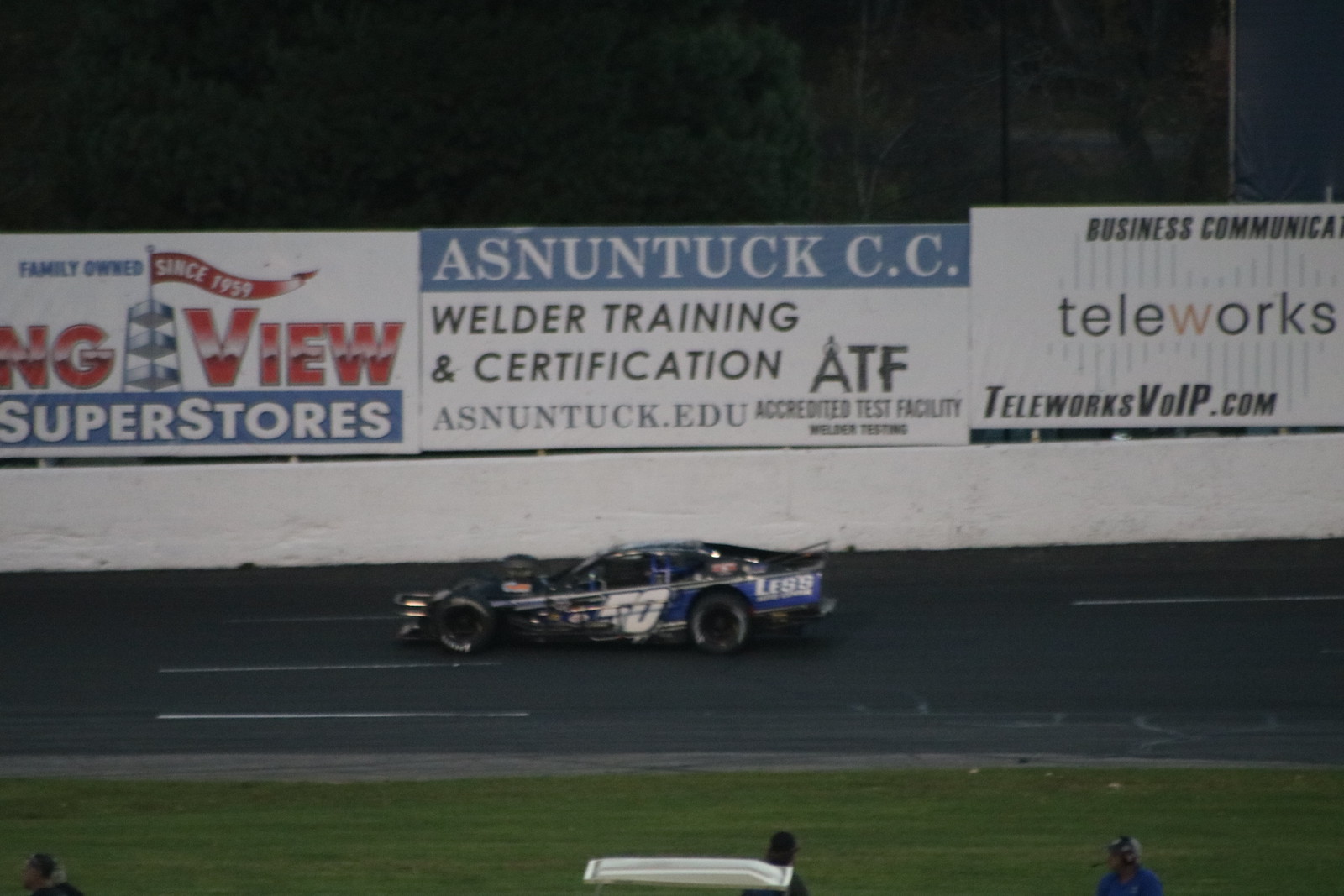Under dim lighting conditions, possibly at dusk or nighttime, this image captures a dynamic scene at a racetrack. The focal point of the photograph is a black stock car with a striking blue stripe running along the driver's side, prominently featuring the number 50 in white on its door. The car, possibly powered by a V8 engine, sports thick Goodyear tires. In the foreground, three crew pit members are visible, their backs turned to the camera as they stand near the grassy infield, adding to the action and realism of the event. Across the track, there is a white retaining wall, marked by scuffs from previous collisions. Above the wall, several advertisements are displayed, including banners for "Superstores" on the left, "Asnuntuck Community College Welder Training and Certification" in the center, and "Teleworkz VoIP.com" on the right. Beyond the fence, a solitary tree stands silhouetted against the darkened sky, completing the vivid and bustling atmosphere of the racing event.